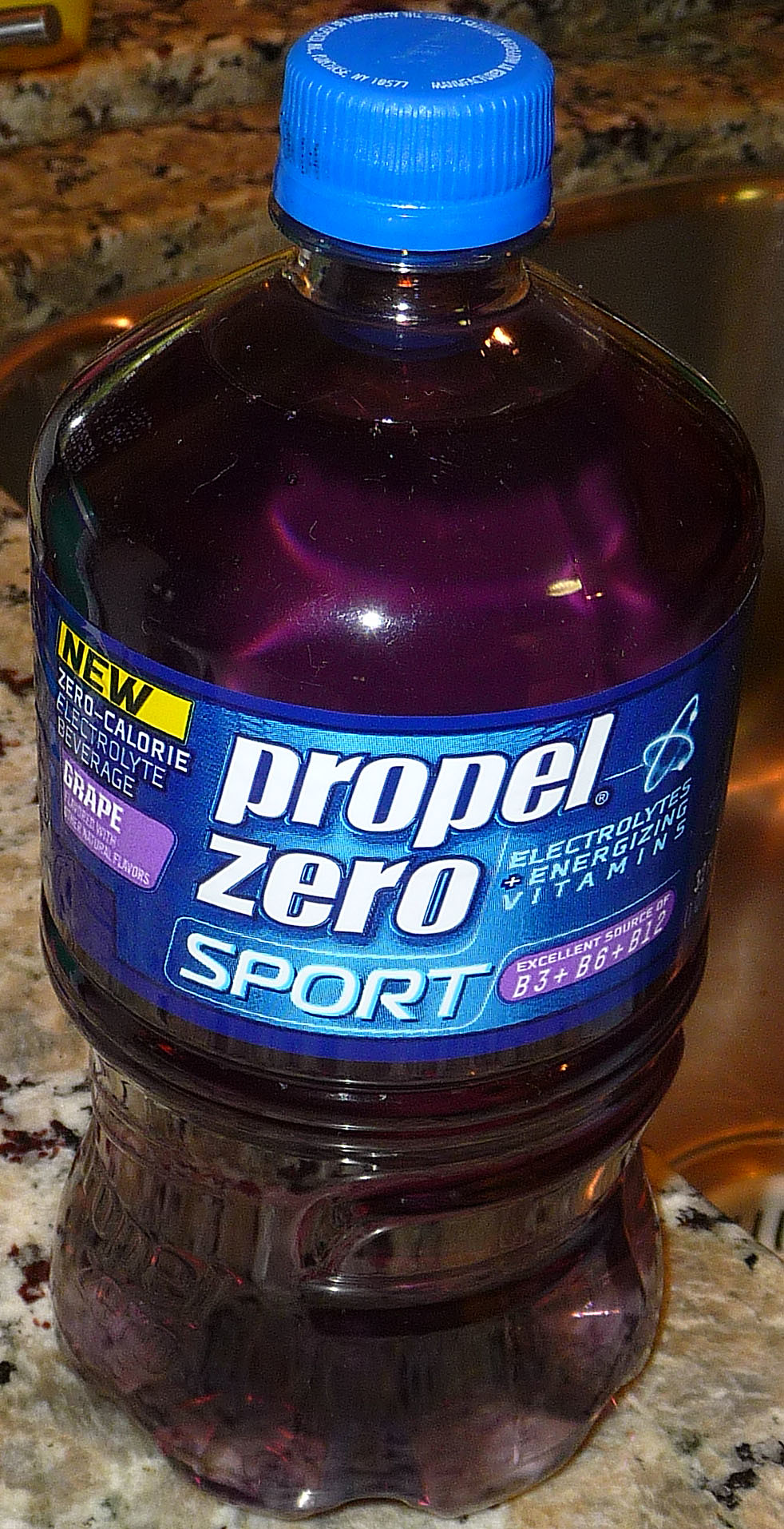This close-up image showcases a bottle of Propel Zero Sport, prominently featuring its distinct blue cap and a blue-themed label with various informational highlights. The clear bottle contains a purple liquid, identified as grape-flavored. The label details that it is a new zero-calorie electrolyte beverage, boasting energizing vitamins. Key information is displayed in white writing against different colored backgrounds: the text "Propel Zero Sport" is prominently featured with dark blue trim, while various nutritional benefits are outlined, including an excellent source of vitamins B3, B6, and B12. The bottle rests on a granite countertop that has a complex pattern of brown, beige, gray, and black, adjacent to a sink and possibly near a copper-colored item.